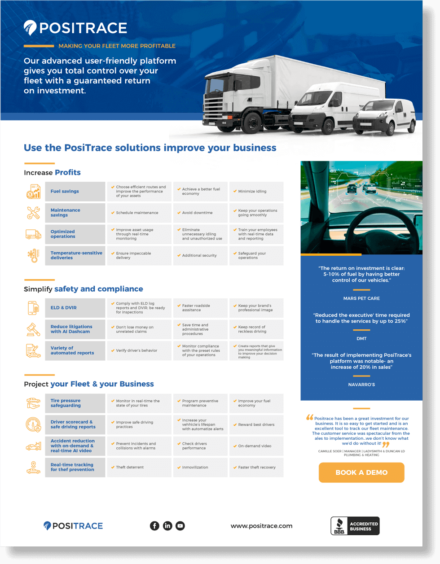**Screenshot of Positrace Fleet Management Service Interface**

This image is a small, low-quality screenshot showcasing the homepage of Positrace, a global fleet management service based in British Columbia. At the top of the page, a blue banner with a faded image of a driver in the background prominently features the Positrace logo and the tagline: "Positrace – Making Your Fleet More Profitable." This text emphasizes the service's promise of an advanced, user-friendly platform that offers total control over your fleet along with a guaranteed return on investment. 

Below the banner are images of three different white vehicles: a semi-truck, a moving van, and a smaller hatchback van, representing diverse fleet types. Moving further down, the page introduces the benefits of Positrace solutions with a headline, albeit with a minor typo, urging businesses to "improve your business" and "increase profits." 

The interface is structured into multiple sections. One detailed area presents a 16-block grid that outlines various advantages of using Positrace, such as fuel savings, maintenance savings, and the management of temperature-sensitive deliveries. Despite the information being difficult to read due to the poor screenshot quality, it provides significant detail about the platform’s functionalities. 

Further down, another section focuses on enhancing safety and compliance through data, displayed in a 12-box grid of benefits. The final section emphasizes the protection of both the fleet and the business, laid out in another 16-box grid describing related positives. 

To the right of these sections, there's a graphic showing a person driving a vehicle, capturing just the steering wheel and the road ahead. Below this image, additional descriptions and a review in quotes provide further insights into the service’s effectiveness. 

At the bottom of the screenshot, there is an orange rectangular box prompting users to "Book a Demo.” Finally, the footer of the page contains the Positrace logo once more, along with icons linking to Facebook, LinkedIn, and another social media platform, as well as an "Accredited Business" badge on the far right.